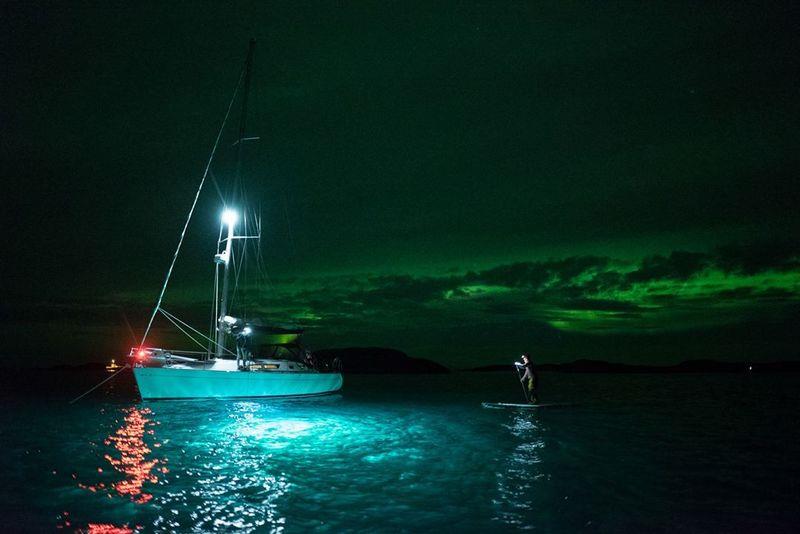This evocative photograph captures the serene scene of an illuminated light blue fishing boat or sailboat, situated slightly to the center left of the image. Taken during the twilight hours of either morning or evening, a gentle glow emanates from a light atop the boat's mast, casting a soothing reflection onto the deep blue and black waters beneath. Adding more to the ambiance, a red light at the bow of the boat contributes another layer of reflection on the water's surface. Behind the boat, a man on a paddleboard appears, identified by a light affixed to his head, adding a subtle human element to the stillness. In the background, distant islands dot the horizon under a sky that transitions from a peculiar black-green hue to almost pitch black directly above the boat, creating a striking and almost otherworldly atmosphere.